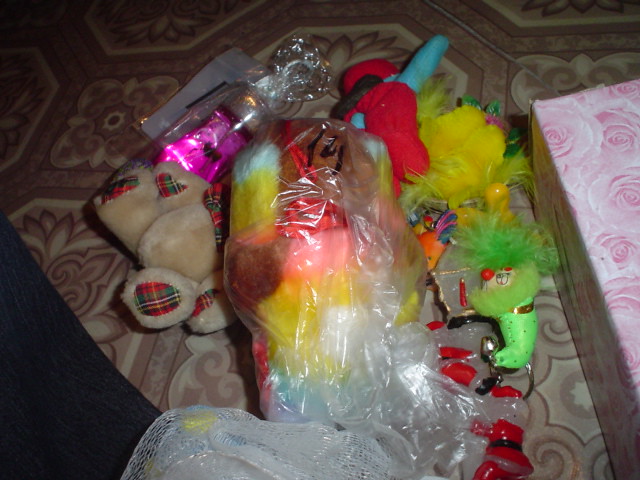The image captures a vibrant and meticulously detailed scene of a children's toy collection. Positioned prominently in the center is a plastic bag brimming with an array of plush toys, including a bear with a white belly and plaid-colored pads on its feet and hands, a yellow furry bird, and a unique green character with a shrimp-like tail and a bell at its end. Surrounding the bag are additional toys in various compositions, some soft and fluffy like the red and white Santa Claus candy toy, and others more rigid and plastic. A distinctive red toy, featuring what appears to be either an arm or a unicorn horn, adds to the assortment.

To the right, a gift box covered in pink and white rose-patterned wrapping paper suggests that these toys have just been unwrapped, perhaps during a celebration. The scene is set on a decorative, patterned carpet in a living room, with colors ranging from light red to beige that complement the light spectrum of hues from the toys. Subtle highlighting on the plastic bag accentuates the textures and suggests the use of a flash in the photograph, giving the entire image a warm and inviting indoor ambiance.